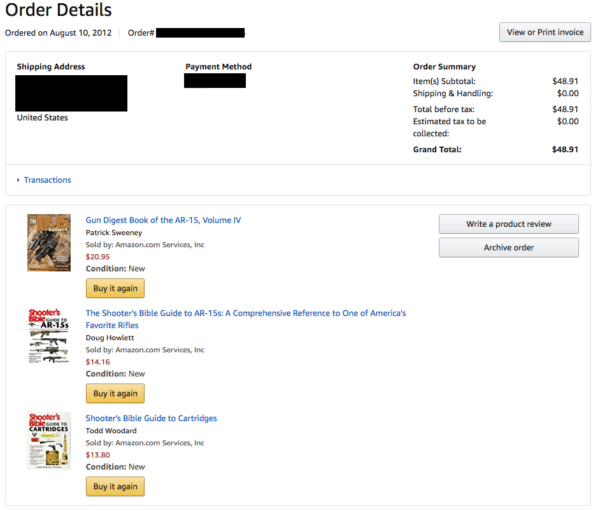**Detailed Caption:**

The image features a screenshot of an e-commerce website, highlighting the "Order Details" section of a purchase receipt. Set against a predominantly white background, the section provides a detailed summary of an order placed on August 10th, 2012. Key elements include an "Order Number" that has been blacked out for privacy and an adjacent button labeled "View or Print Invoice," confirming that this is an online, printable invoice.

On the left side of the screenshot, under the heading "Shipping Address," all specific information has been blacked out except for the fact that the shipment is within the United States. In the same line but towards the center, the "Payment Method" is also obscured.

The order summary displays a subtotal, shipping and handling fees, a total before tax, estimated tax, and a grand total amounting to $48.91. The summary also lists several items purchased, each accompanied by a thumbnail image of the book cover, pricing details, the author's name, and a "Buy Again" button. The items include "Gun Digest Book of The AR," "Shooter's Bible Guide to AR-15," and "Shooter's Bible Guide to Cartridges."